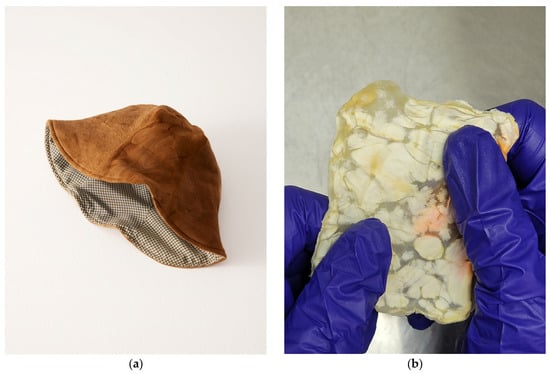The image consists of two adjacent pictures labeled "A" and "B." On the left, picture A features a medium brown baby cap with a wave-shaped lower border. Its texture appears soft and slightly wrinkled, and the inside is lined with a green and white gingham check pattern. The background of this picture is a plain white. On the right, picture B shows a person wearing latex gloves—blue on one hand and purple on the other—against a gray backdrop. The hands are outstretching a package that appears to be wrapped in plastic and has a textured, white surface. The overall color palette includes brown, light grayish white, gray, beige, off-yellow, purple, and darker gray. There is no text present in either of the images.